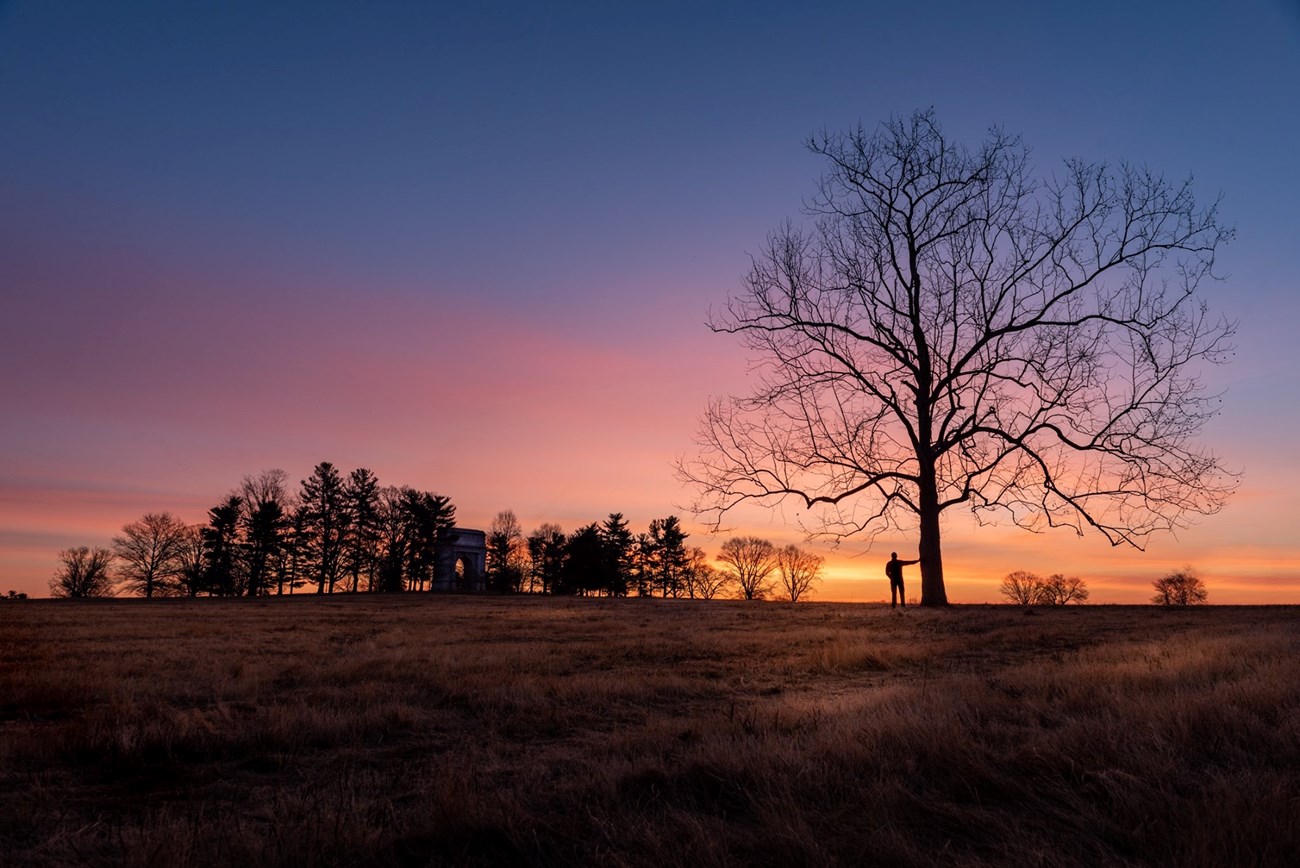In this captivating photograph taken at sunset, a man is depicted as a tiny silhouette leaning against a colossal tree, highlighting the immense scale difference between him and the towering trunk. His arm is outstretched, pressing against the tree as he gazes at the breathtaking sunset. The sky is a stunning blend of colors, transitioning from deep blue at the top through shades of purple, pink, and orange, down to a mix of dark and light blue near the horizon. The foreground features an open, brown field with tall, wispy, straw-colored grass that adds texture to the scene. In the distance, additional trees and maybe even a silo or a house can be faintly seen, standing amongst more trees, contributing to the picturesque composition. The overall atmosphere suggests a tranquil moment either early in the morning or, more likely, at the closing of a slightly cloudy day in the fall, with the vivid colors of the sunset dominating the visual narrative of the image.